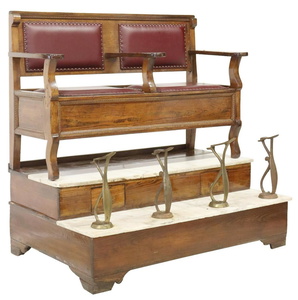The photograph showcases an intricately designed, antique shoe-shining bench made entirely of dark brown wood. The bench is multi-tiered, featuring a lower step and an elevated seating area. The seat, designed for two individuals, is adorned with rich mahogany cushions for both the seating area and backrest, offering comfort and support. This particular bench also includes three armrests, two on each side and one in the middle, emphasizing its capacity to accommodate two people simultaneously. The lower tier of the bench features protruding metal stirrups, slightly curved to fit the natural shape of the feet, enabling patrons to place their feet up while their shoes are detailed and shined. The entire piece is set against a pure white background, highlighting its detailed craftsmanship and design, and suggesting its use as a functional, yet visually appealing, antique furniture item.